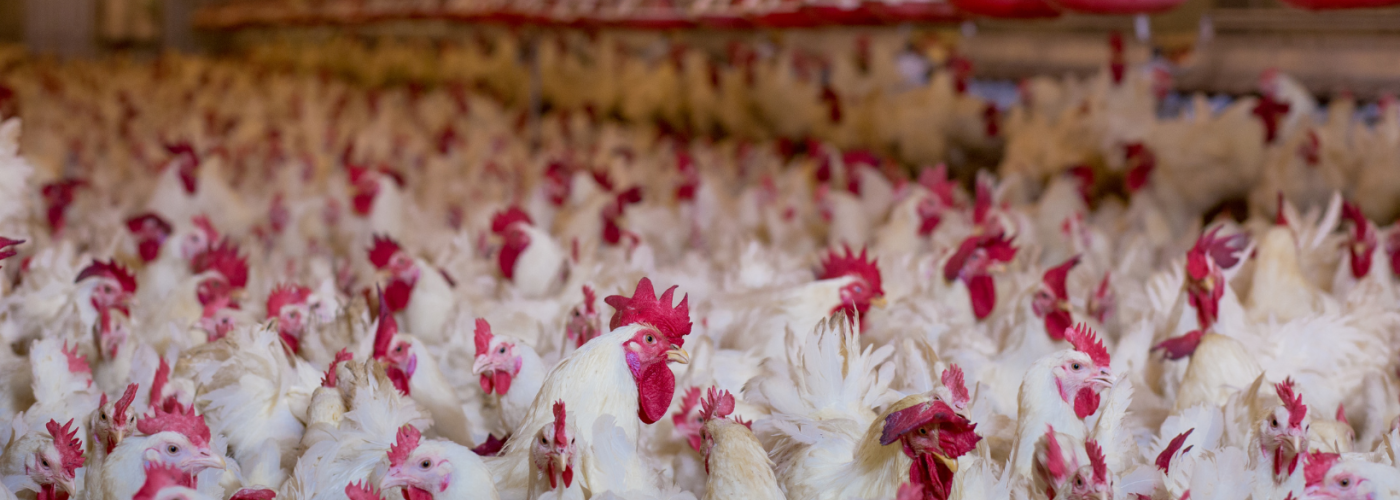This is a wide, horizontally aligned panoramic photograph capturing a vast room filled with hundreds of nearly identical white feathered roosters. Each rooster features a red comb atop its head, red wattles beneath its beak, and small black eyes. The heads, especially in the foreground, are meticulously detailed, showcasing the vibrant contrast between their white bodies and the red around their eyes and crowns. In the foreground, the focus is sharp, revealing the intricate patterns and textures of their feathers and facial features. As the image extends into the background, a blur takes over, hinting at the countless more roosters stretching deep into the distance. A subtle gap runs from the lower right to the upper left, and on the upper right-hand side, the edge of a wall is faintly visible. The beaks vary slightly in color, exhibiting shades of yellow or tan. This densely packed scene of roosters creates an almost overwhelming sea of white feathers punctuated by striking red accents.